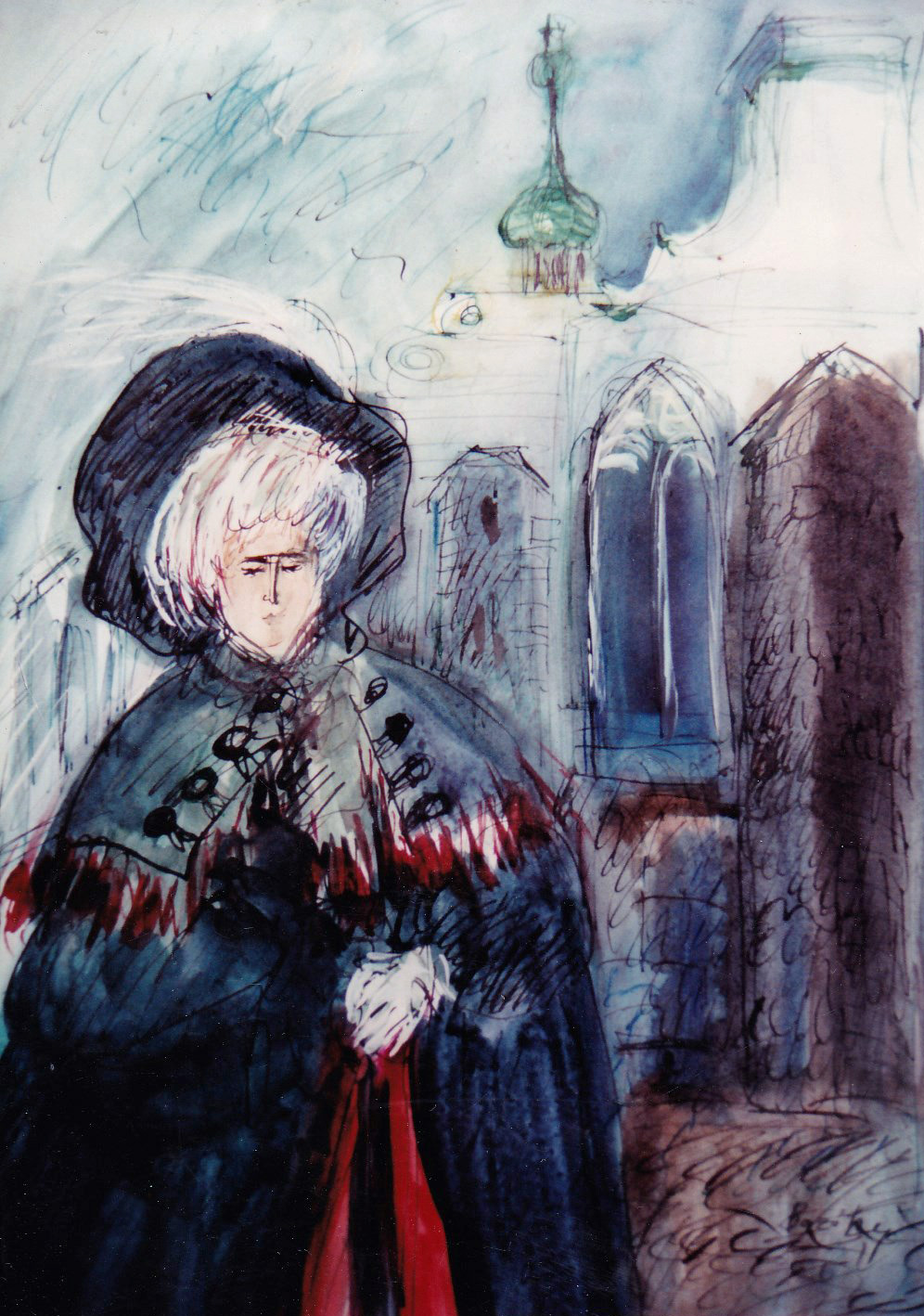The image is a highly detailed drawing, possibly incorporating both pen and oil paint, depicting an older woman with large white hair. She is adorned in a regal attire consisting of a dark blue and black robe with inner red linings, and a gray shawl draped over her shoulders. Her elaborate headdress resembles an old-style bonnet, adding to her stately appearance. The woman wears white gloves and clasps her hands in front of her, exuding an air of attentiveness. Behind her, a majestic stone building with a cathedral-like architecture rises, featuring pointed, turquoise-tinted spires and traditional arched doors. The background captures a textured sky, variably patched with white and blue, enhancing the scene's grandeur. Additionally, the scene includes a brown stone column and what appears to be a light fixture or chandelier hanging from the ceiling, indicating an indoor setting that blends with the external cathedral backdrop.